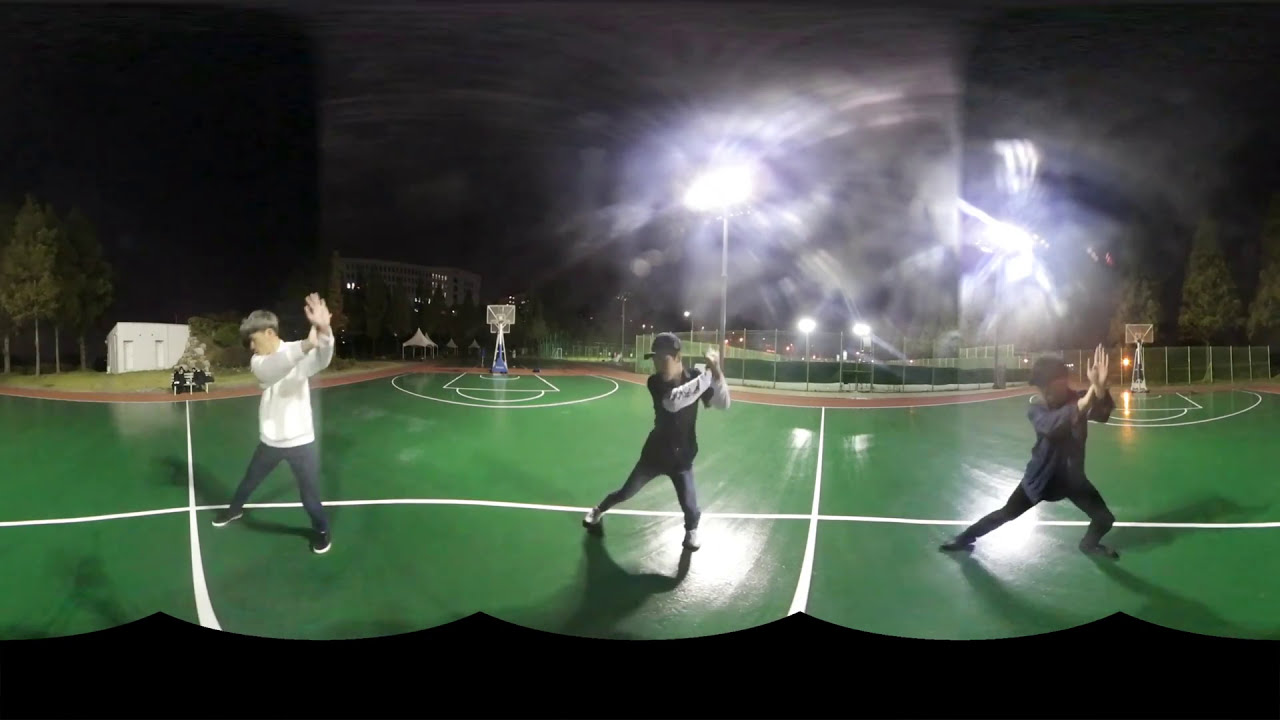In this stitched image, we're viewing three young men on a green basketball court at nighttime, illuminated by several bright lights. The curvy wave along the bottom reveals that the scene has been captured using multiple lenses. The boys appear to be dancing or practicing martial arts, each striking a dynamic pose. Starting from the left, the first boy, who has blonde hair and is Caucasian, wears a white jacket and black pants. He raises his left arm towards the sky with his right arm supporting it. Positioned to his right, the second boy wears a black baseball cap, a black short-sleeved shirt with white sleeves, and gray sweatpants. His arms are similarly raised, but less outstretched. Finally, the third boy dons a navy blue jacket with black pants, extending his arm towards the viewer with more stretched-out legs. The basketball court is surrounded by a red running track and features white lines on its surface. In the background, pine trees and a small tent are visible under the dark sky, which adds to the atmosphere of the nighttime scene.